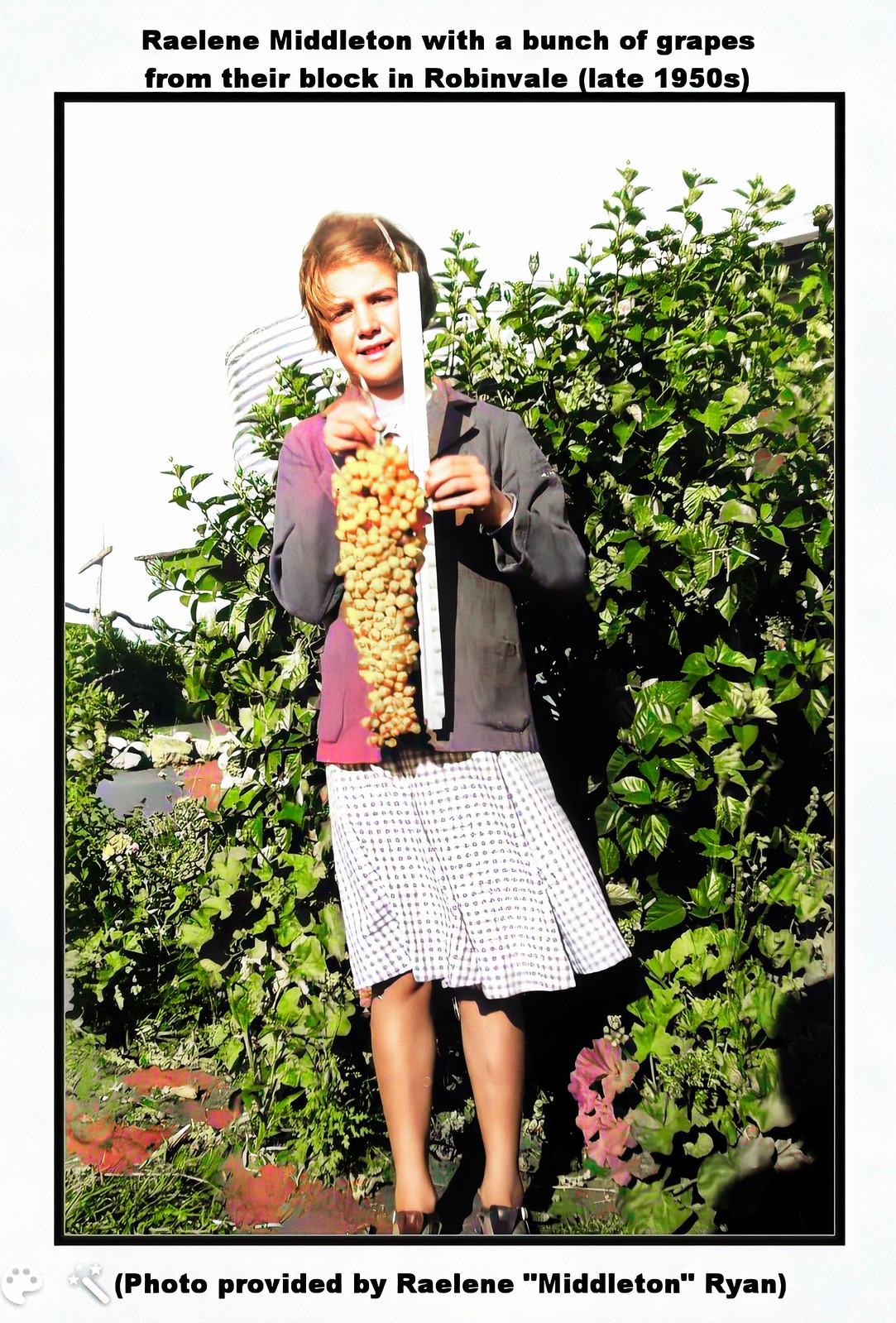This vintage 1950s color photograph showcases a young girl named Raylene Middleton, captured in their outdoor garden in Robinvale. She is standing in front of a lush green bush bathed in sunlight, suggesting the photo was taken during the day. Raylene has short blonde hair and is dressed in a white dotted frock paired with a distinctive grey and pink colored jacket. In her left hand, she holds a white ruler, while her right hand carries a bunch of grapes, a mix of green and darker ones. The image is bordered in black and set against a light grey background, with additional artistic logos in the bottom left corner. The top of the photo features the caption, "Raylene Middleton with a bunch of grapes from their block in Robinvale, late 1950s," indicating the date and location, while the bottom credits the source: "(Photo provided by Raylene Middleton Ryan)." A shadow in the bottom right corner reveals the presence of the photographer.